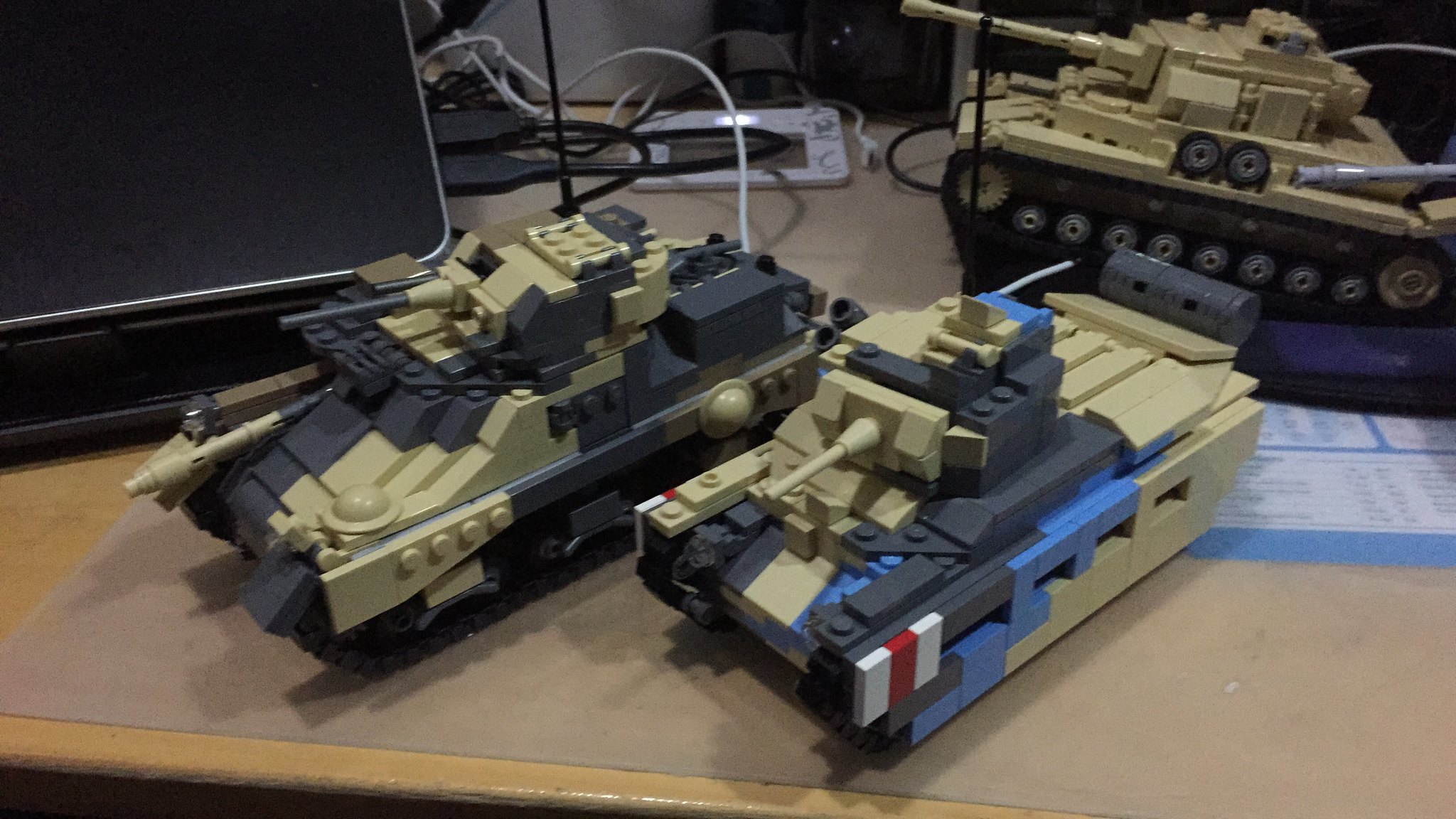This color photograph showcases three army toy tanks made from Lego-style pieces, positioned on a light brown wooden table. The models feature light olive green as their base color, with black accents on top and turquoise blue highlights along the right side. Scattered white and red blocks add additional contrast. The tanks, two facing west and one facing east, differ slightly in color scheme with some parts appearing grayish or light khaki green. Also visible in the image is a sheet of beige paper on the table and a black computer monitor screen in the top left corner. A tangled web of cords can be seen in the background, hinting at a cluttered desk environment.